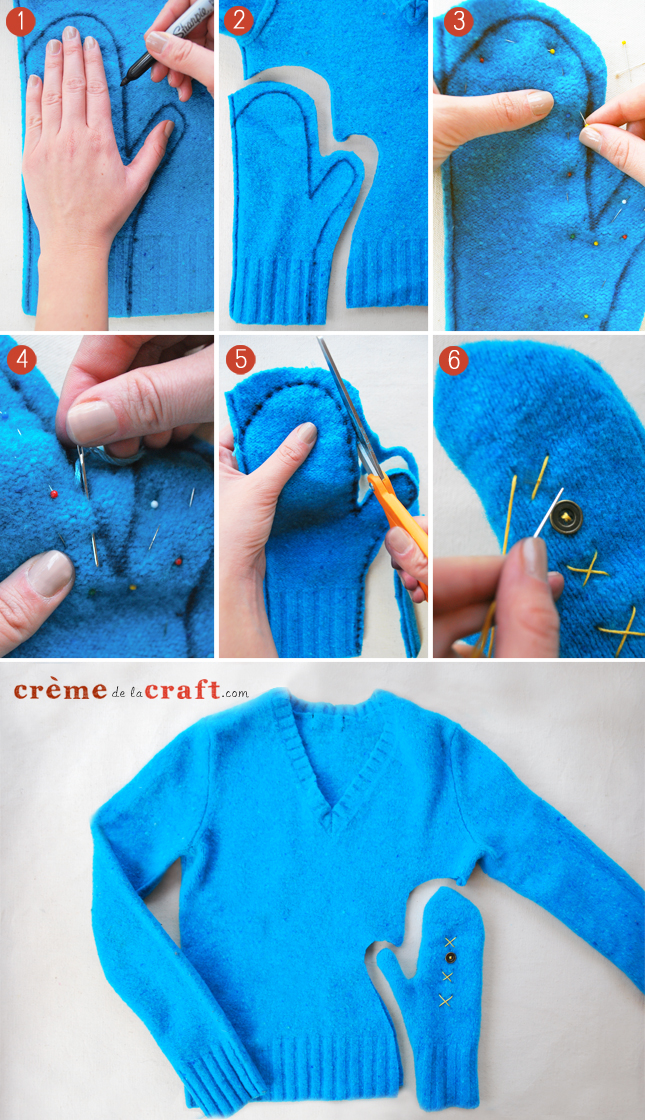The image depicts a step-by-step guide for creating mittens from a blue v-neck sweater, as featured on cremedelacraft.com. The process is illustrated across six stages, starting with tracing a left hand onto the sweater with a marker. The next step shows cutting out the hand-shaped outline from the sweater. In the third step, the cut fabric is pinned together in preparation for sewing. The fourth image displays the actual sewing of the fabric to form the mitten shape, while the fifth step involves trimming the excess fabric around the sewn outline. In the final step, final touches, including sewing small designs and attaching a button to the top of the mittens, are added. The bottom portion of the image highlights the blue sweater with a mitten cut-out, emphasizing the source of the project.